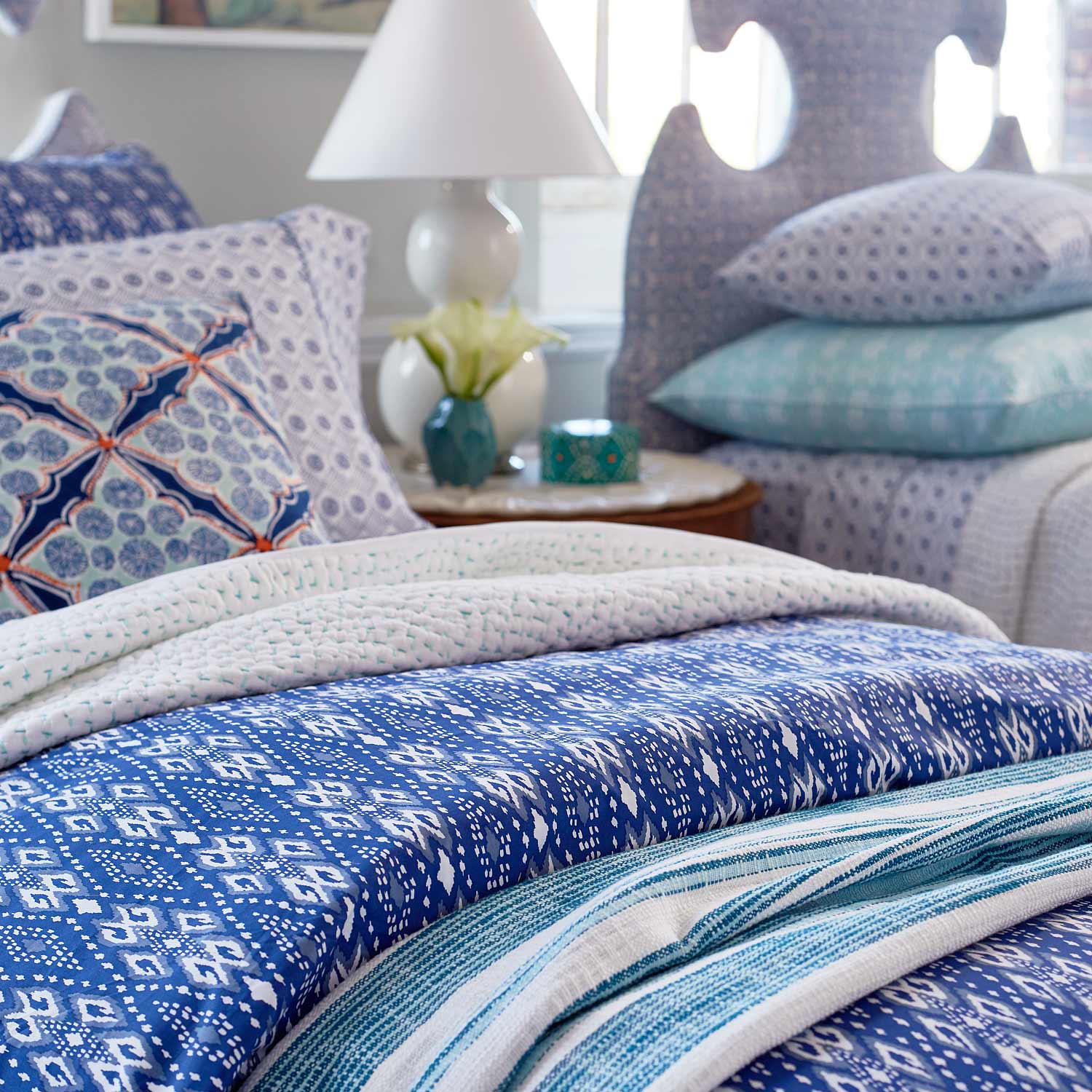This detailed image showcases a bright, modern bedroom featuring two comfortable beds with an emphasis on a blue and white color scheme. The lower left corner of the image highlights a larger bed draped with various blankets and pillows. The bedding includes a blue and white striped blanket, complemented by a white knitted throw folded over a blue and white comforter. Pillows on this bed range in designs, including a dark blue pillow, a white one with blue dots, and another white pillow adorned with a blue print, all contributing to a layered, plush look.

The upper right corner reveals a second bed, partially in view, topped with large, fluffy white pillows and a beige headboard. Both beds share several design elements: thick blankets, numerous pillows, and a mix of patterns creating a cohesive aesthetic. 

Situated between the two beds, a nightstand holds a white lamp with a distinctive large white lampshade and two white spherical accents beneath it. Other objects, including a small green vase, are placed atop the nightstand. The room benefits from abundant natural light streaming in through a window behind the second bed, enhancing the clean and inviting atmosphere. Beige walls provide a neutral backdrop, allowing the blue and white textiles to stand out and create a serene, cozy environment.